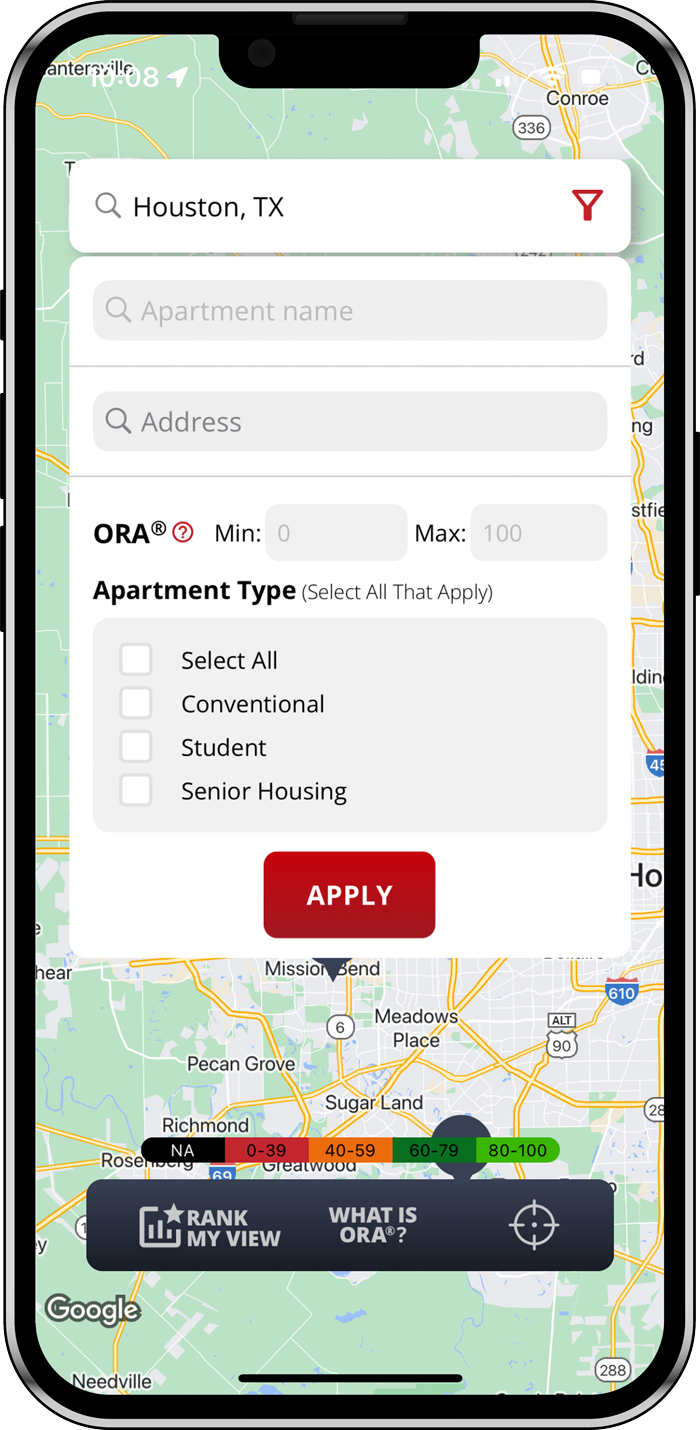This detailed mock-up showcases a smartphone displaying a map application. At the top of the app, there is a search bar with the text "Houston, TX." To the right of the search bar, a filter icon is prominently visible. Directly below the search bar, a labeled field prompts the user to "search for a partner name." Beneath this, there is an address input section. Further down, the interface features a section labeled "ORA," including a small registered trademark symbol (®) next to it. Just above this section, a help icon, represented by a question mark, can be found. Towards the bottom of the display, there is a range slider with the minimum value set to zero and the maximum value at one hundred men.